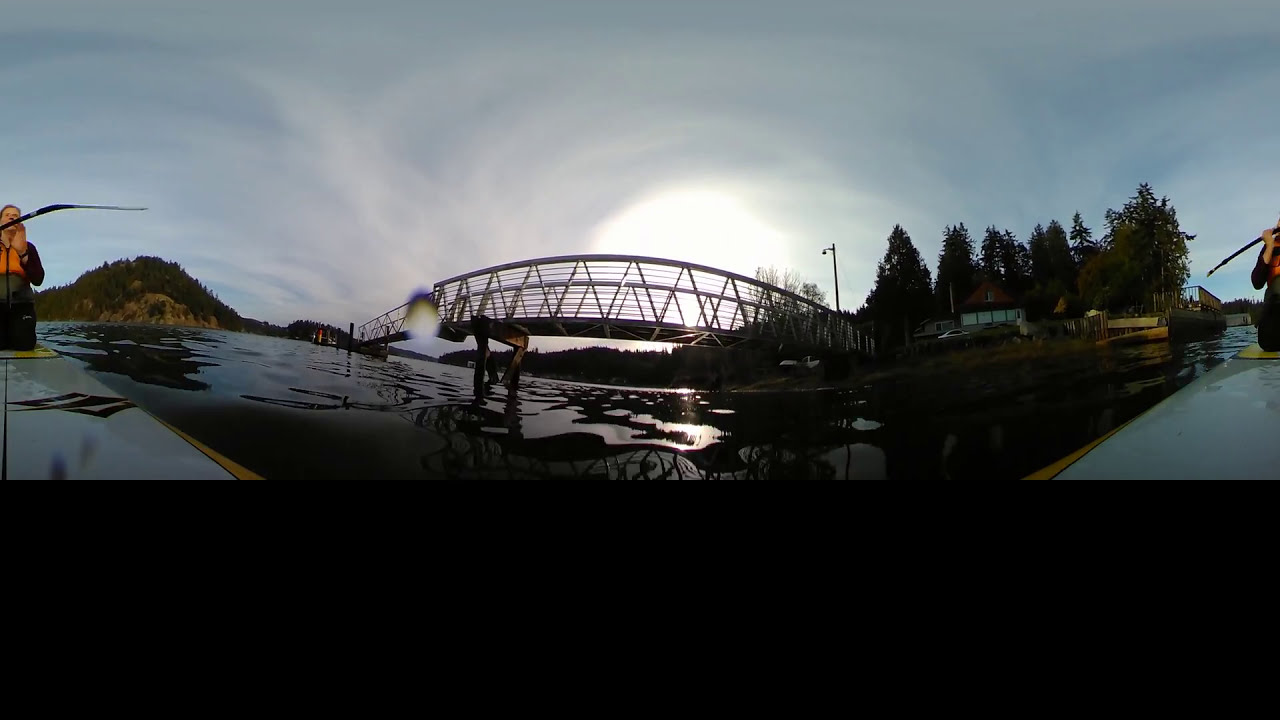This 360-degree image captures a wide-angle view of a serene water body, likely an ocean or a river, framed by a long, intricate bridge above. The bridge, extending from left to right, features a distinctive triangular pattern on its railings. Positioned on a light gray kayak with black markings and yellow trim, the central figure, wearing an orange life vest and dark clothing, holds a paddle. To the left of this person, there's an island adorned with lush trees, while another lush island with a blue and brown wooden building and tall trees lies to the right. The calm water reflects the stillness of the moment as the sun peers over the bridge, casting its light through the smudged skyline dotted with clouds. A yellow boat can also be seen docked next to the land on the right.